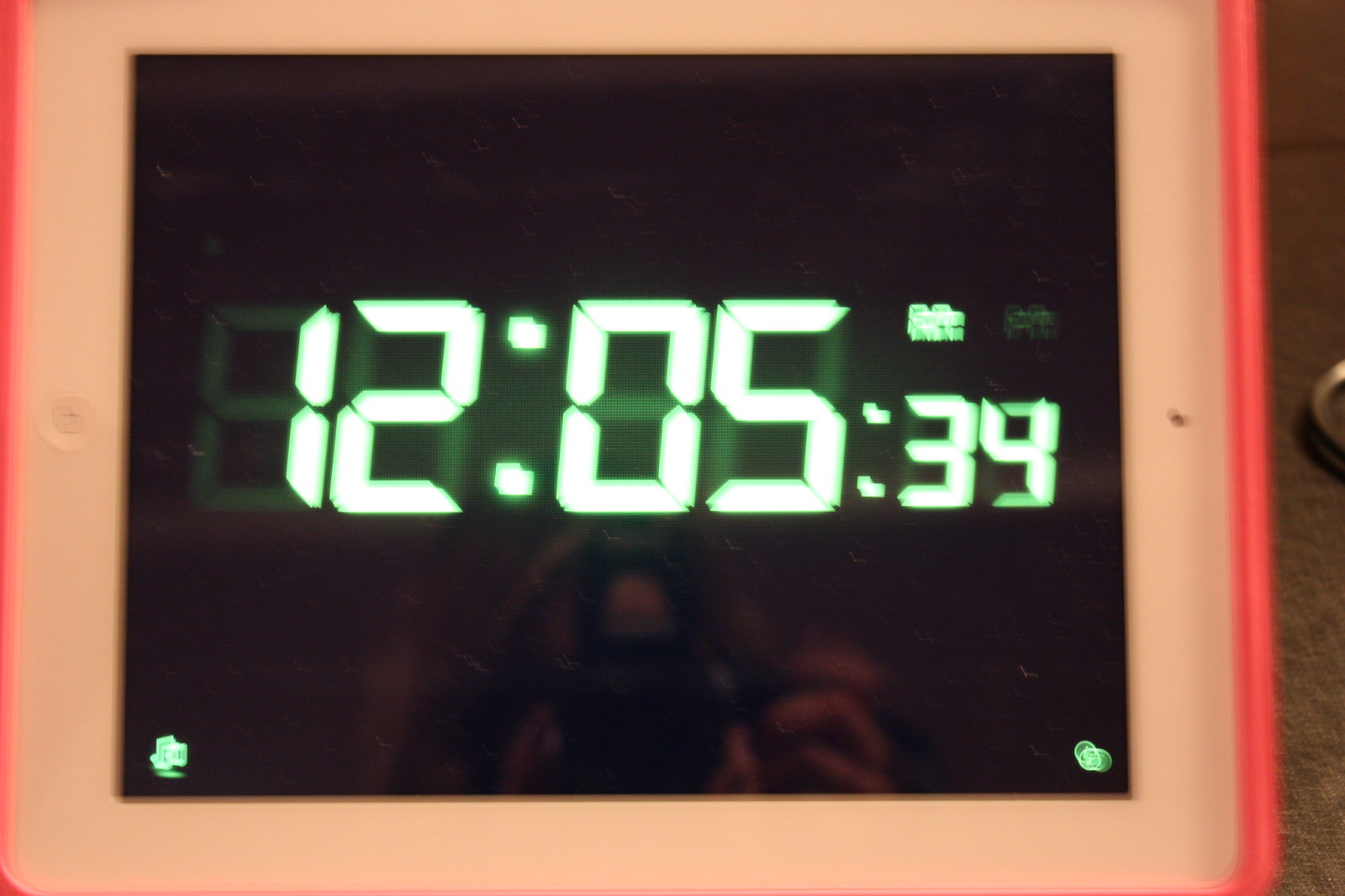A digital alarm clock is at the center of this photograph. The clock display reads "12:05:34" in bright green digital numbers, though it is unclear whether it is AM or PM. The clock resembles a tablet, possibly an iPad, due to its thick white border and the pink silicone case enveloping it. The screen of the clock is black and faintly reflective, capturing the silhouette of the photographer holding a camera with a flash attachment on top. The flash did not activate, leaving the lighting natural. The setting appears to be a bedroom or living room, though there are no discernible background details to provide context.